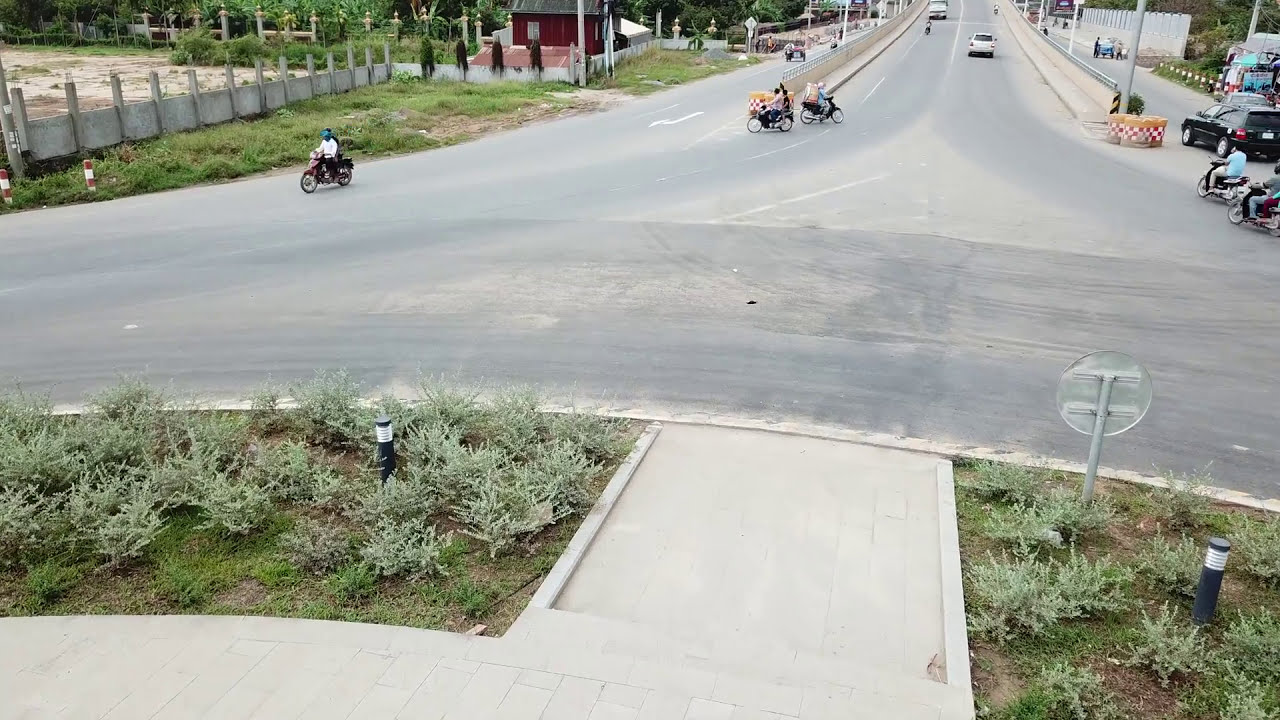The image depicts a busy roundabout with a road intersecting it prominently in the middle and extending towards the top of the frame. Several motorized bikes, two of which are carrying loads that resemble groceries, are visible on the road. There are also multiple cars on the road, including a black car to the right and a couple of white cars traveling down the center. The bottom part of the image features a light white brick sidewalk, accompanied by sparse, short shrubs and bushes. To the upper left corner, there is a sandy area bordered by a gray cement brick barrier. At the very top of the picture, a red barn can be seen. The scene includes landscaped green foliage around the roundabout and a small fence or posts positioned to prevent vehicle entry, contributing to the overall busyness and functionality of the street environment.